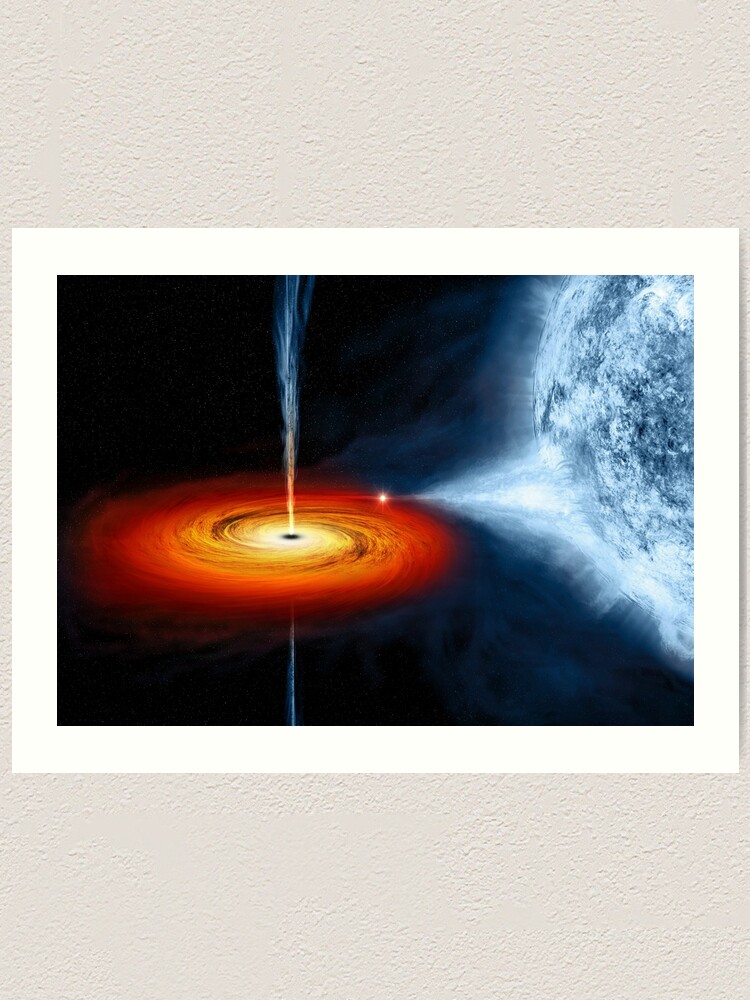The photo captures a poster displayed on a beige wall, featuring a spectacular astronomical phenomenon. The poster's central image vividly portrays a massive black hole situated left-center, surrounded by swirling bands of matter in successive layers of white, yellow, and orange. Emanating vertically from the black hole are luminous jets of radiation—Hawking radiation—extending above and below the black hole. The upward jet transitions from yellow at the base to blue as it ascends off the top of the image, while a similar blue stream emerges downward, disappearing off the bottom edge. On the right side of the image, the chaotic scene includes a smaller celestial object being drawn into the black hole's gravitational pull, possibly remnants of a Sun-like star ejecting into the surrounding space. This dynamic scene is set against the backdrop of a blue-tinged planetary body at the upper right, depicted with curving edges that give it a near whirling appearance, emphasizing the pervasive influence of the black hole's gravity. The poster itself is framed by a thick gray border on the top and bottom, with a thin white border encasing the vivid scene, making the stunning celestial display pop against the minimalist wall.